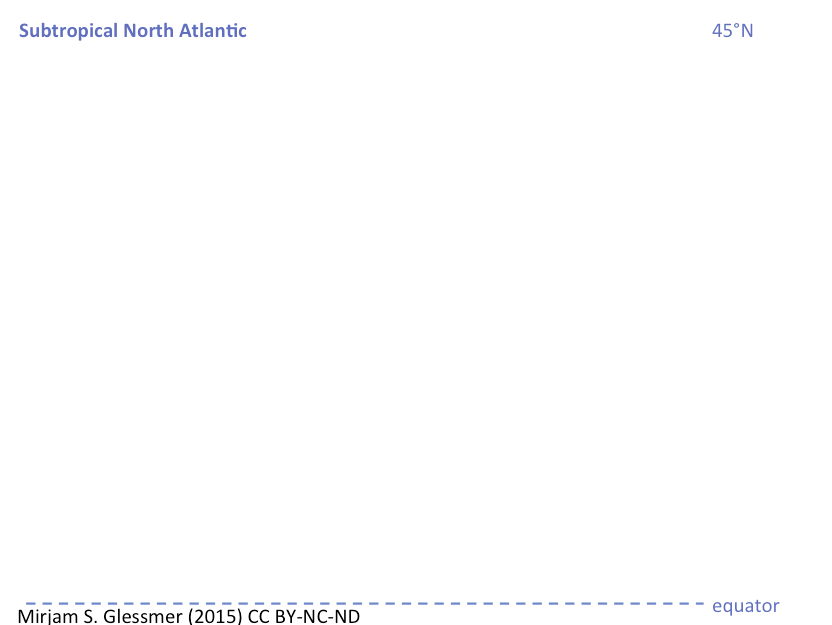A webpage with minimalistic design features: At the top left corner, blue text reads "Subtropical North Atlantic." On the top right, it displays "45°N" in blue font. The majority of the page is blank with a white background. At the very bottom, a horizontal dashed blue line stretches across the page. Positioned at the lower right corner beside this line, the word "Equator" appears in blue text. Below the dashed line on the left, the author's name, "Mirjam S. Glessmer (2015)," is marked in black. Adjacent to this, the licensing information "CC BY-NC-ND" is written in uppercase. These are all the elements on the page, with no additional content or imagery present.